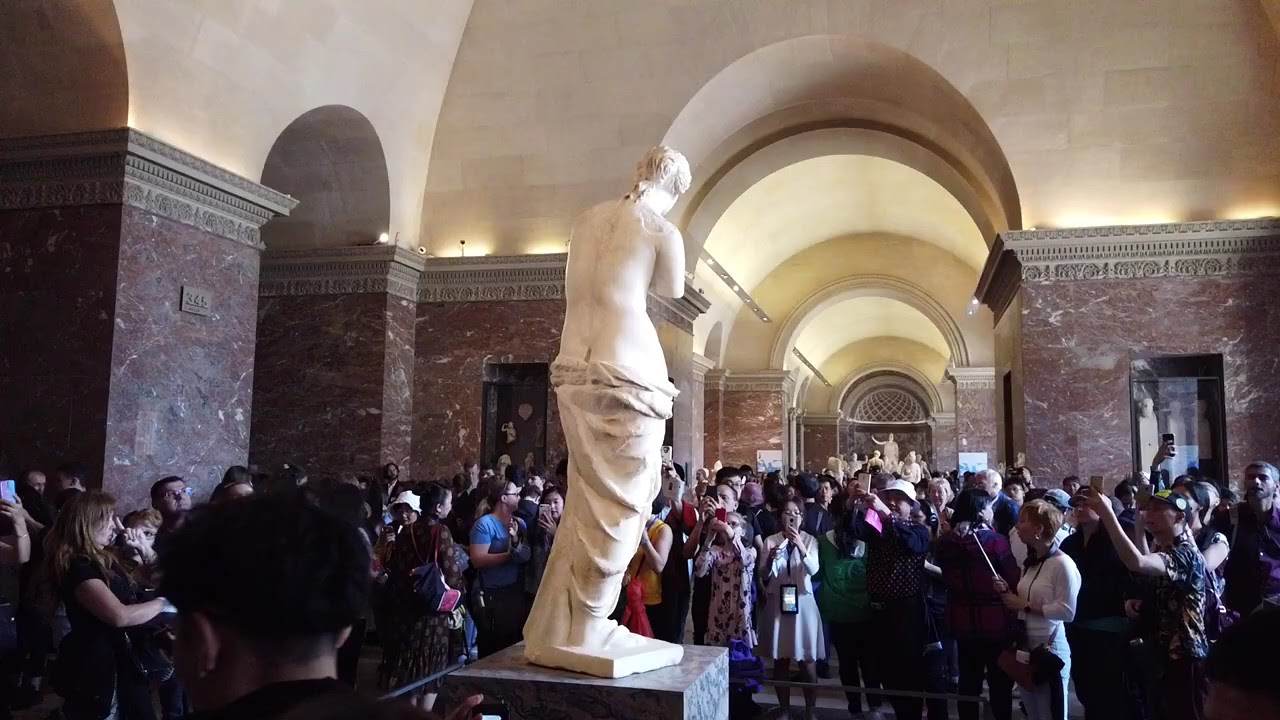The color photograph captures the grand interior of an art gallery or museum, potentially European. At the center stands a detailed, larger-than-life marble statue of a white woman with an ancient, armless form, draped in a garment from the waist down. This female figure rests on a gray square marble platform, around which crowds of visitors gather, many taking photos from various angles. The well-lit, spacious room boasts elegant architectural features, including sloped archways and decadent pillars. The upper sections of the walls are adorned with gray-beige marble, while the lower parts exhibit a rich burgundy streaked marble, contributing to the luxurious ambiance. The hall's ceiling is beige, enhancing the opulent feel, with additional art pieces encased in glass scattered throughout the gallery. This detailed scene is captured in a landscape orientation photograph with a strong sense of realism.